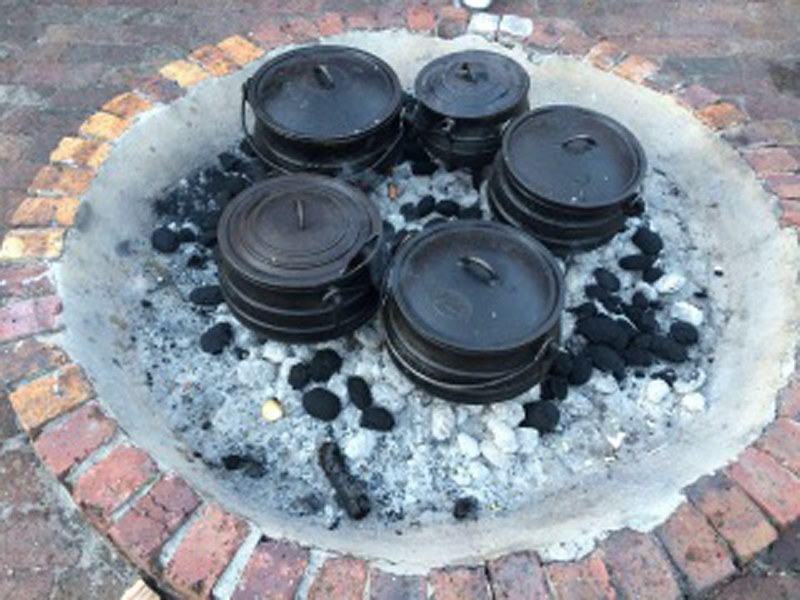This photograph features a large fire pit with a circular brick border, lined with red and orange bricks. The pit itself has a cement bowl shape, creating a spacious interior. Within the pit, there are five large, black cast iron cauldrons arranged in a circular pattern with space in the middle. The cauldrons are characterized by cylindrical shapes and have lids equipped with central handles, as well as long handles on their sides, presumably for carrying. Inside the fire pit, various pieces of white ash and black solid charcoal are scattered, some looking quite spent. The ground inside the pit appears to be covered in a mixture of ash and charcoal. The fire pit is placed on a stone foundation, which extends beyond the border, forming a larger brick-laid area surrounding the structure. The detailed arrangement and elements suggest a well-used, robust cooking setup.